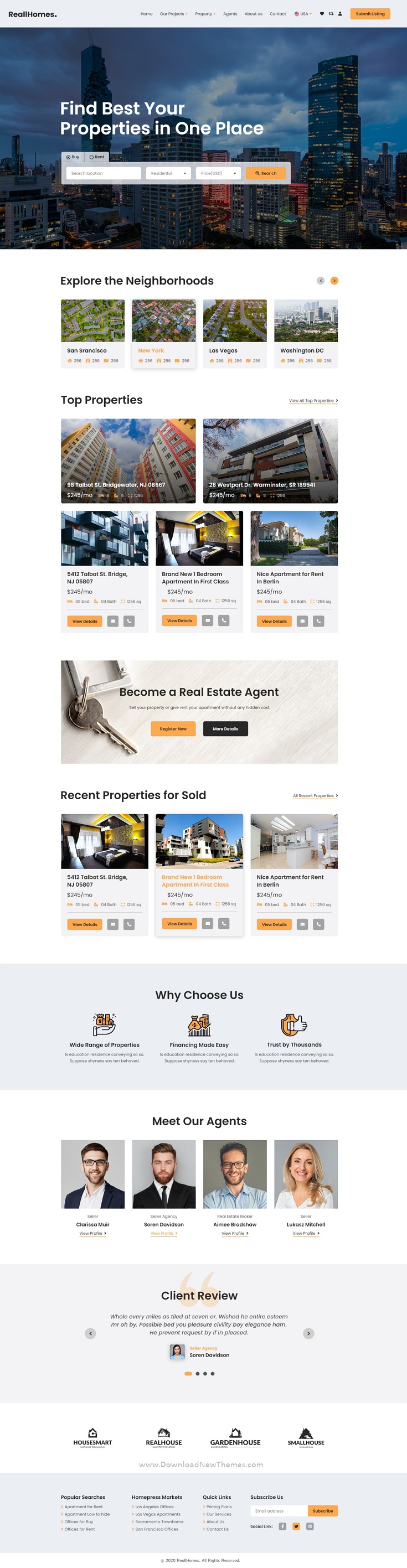In this screenshot, we are looking at a vertically extended webpage with small, slightly blurry text. At the top, a gray header features black text in the upper left corner that reads "Real Homes." To the right, there is a menu in small gray text with the following options: Home, Our Projects, Property, Agents, About Us, Contact, and USA, with a dropdown arrow beside it. In the upper right corner, an orange action button labeled "Submit Listing" is visible. Below the header, a city skyline captured at dusk or dawn spans the width of the image. Bold white text overlays this skyline, stating "Find Your Best Properties in One Place." Near the bottom of the webpage are four headshots of young adults, presumably in their 20s or 30s. Above the photos, black text reads "Meet Our Agents." From left to right, the agents are: Clarissa Moir, Soren Davidson (a young man with a beard, mustache, and brown hair), Amy Bradshaw (a man with a mustache, beard, brown hair, and glasses), and Lucas Mitchell (a young blonde woman wearing a white shirt).